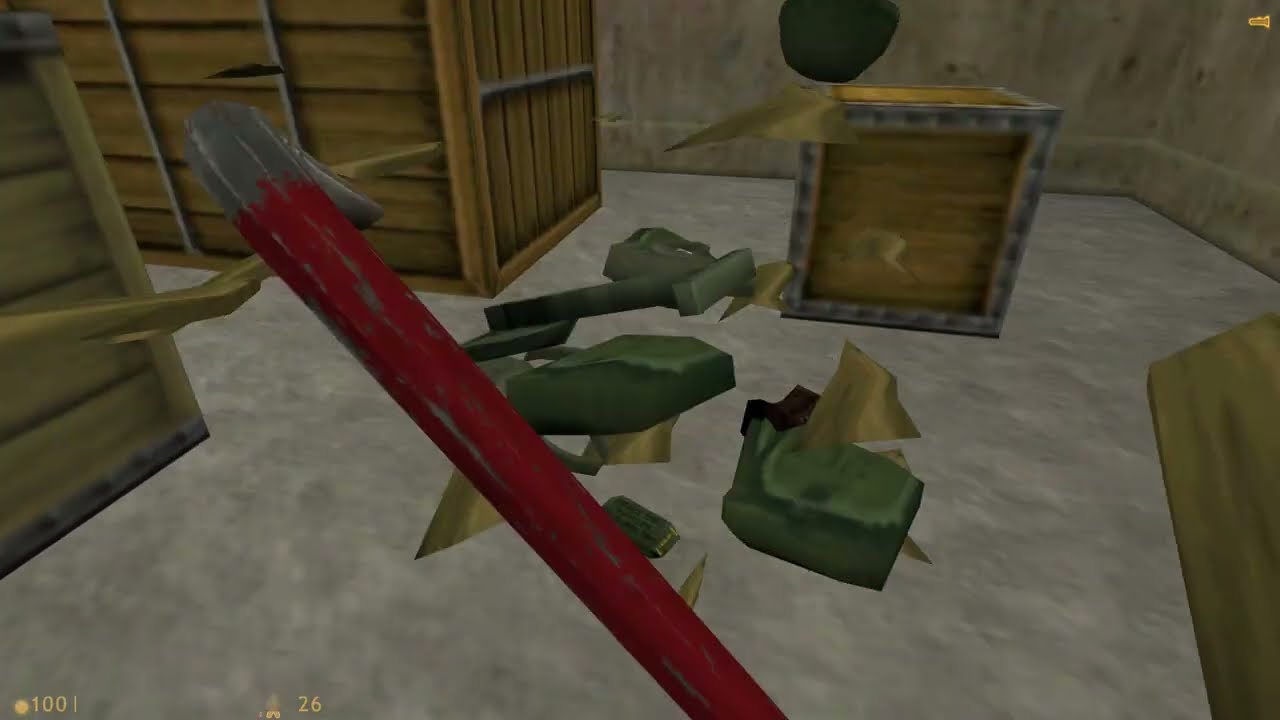This is a screenshot from a video game, showcasing a first-person perspective inside a storage room or warehouse. The scene features grayish light brown concrete floors and slightly darker brown concrete walls. In the upper left corner, there are two large, bright brown wooden crates reinforced with both horizontal and vertical wooden planks. The upper right corner contains a cubic crate with metal borders. Dominating the foreground is a red crowbar with a silver tip, positioned as if it is being held by the player. Scattered on the floor in front of the crowbar are various green and gold items, possibly loot including a shotgun, backpack, and some ammunition. The overall ambiance of the room is characterized by a mix of stone and wooden textures, depicting a typical video game environment filled with crates and scattered items.